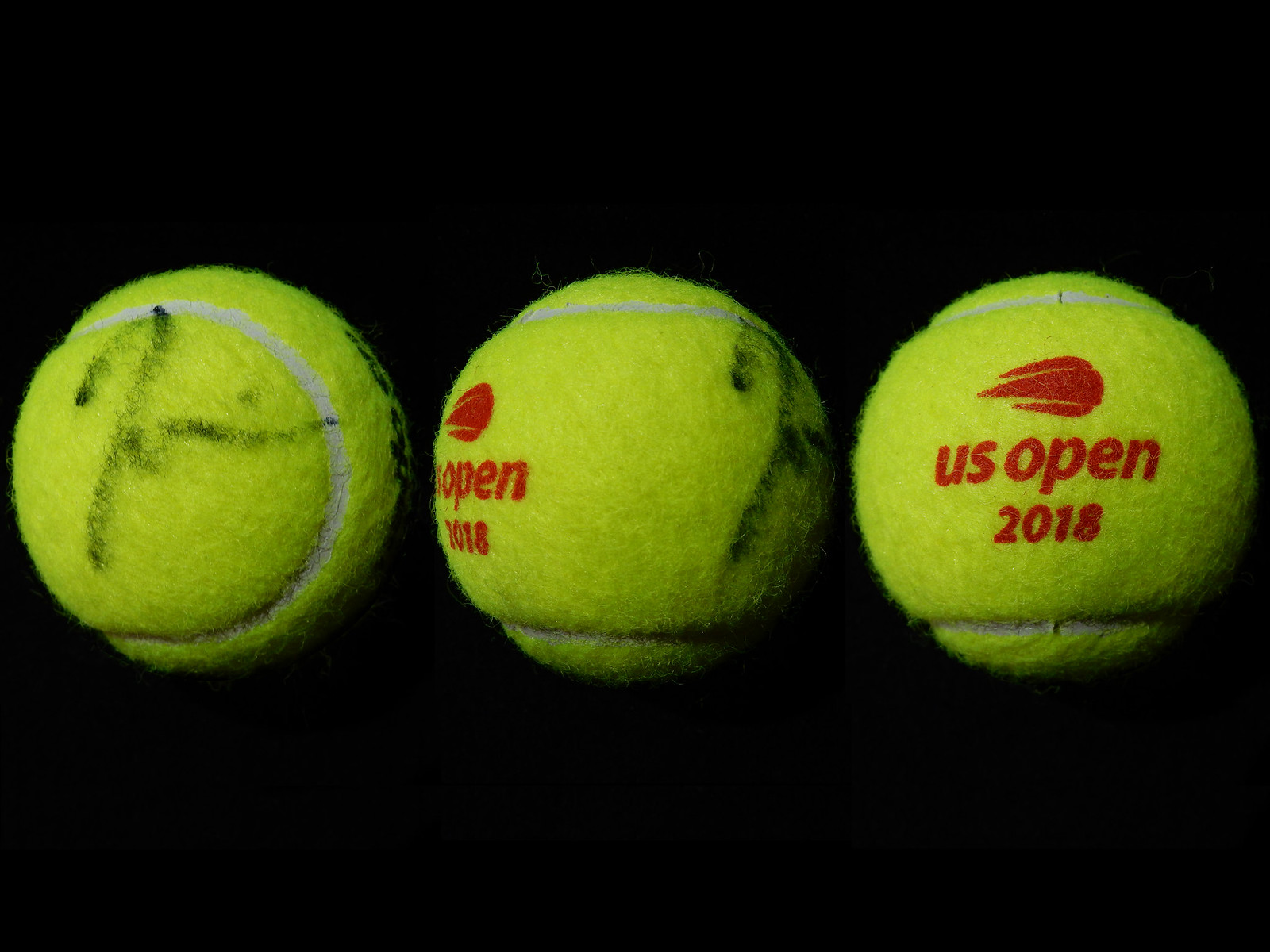This image features three lime green U.S. Open 2018 tennis balls set against a solid black background. From left to right, each ball is positioned to showcase distinct aspects. 

The tennis ball on the left is turned to reveal its white stitching creating a smaller circle within which a faint signature in black marker is visible. Beside it, the middle tennis ball is oriented to partly display both the signature continuing near the edge and a partially obscured red U.S. Open 2018 logo featuring a stylized tennis ball with a three-pronged tail indicative of motion. The tennis ball on the right is positioned to prominently exhibit the full red U.S. Open 2018 logo, although the signature is not visible from this angle. 

This composition likely aims to provide a comprehensive view of the tennis balls, potentially for auction purposes by showcasing all significant details including autographs and logos.